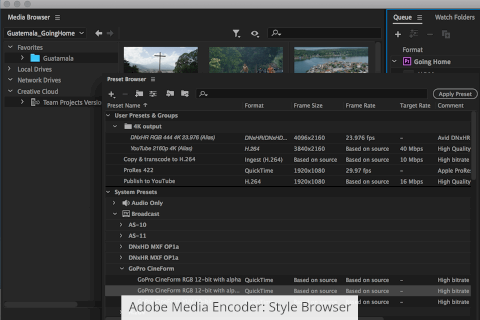The image appears to be a screenshot of a website interface related to media management, likely for organizing and editing multimedia like movies and photos. Due to the image being shrunk, the text and visuals are somewhat blurry. On the left, there’s a label "Media Browser" with a three-line menu icon next to it.

The main content shows a dropdown menu with items such as "Guatemala," "score," and "Gonghei." Below that, the left-hand navigation menu lists different categories. The "Feature Favorites" section displays a folder named "Guatemala," which seemingly contains several pictures. There are also options for "Local Drives," "Network Drives," and "Creative Cloud." Within the Creative Cloud section, there's a nested menu item named "Team Projects Version."

Three preview images are visible: one clearly depicts the Christ the Redeemer statue in Brazil, while the other two are too blurry to make out. Additional icons include a plus sign and multiple folder icons with plus signs, suggesting options to add new content or folders. There is a search bar labeled "Apply Preset," flanked by categorized folders such as "Uses and Presets," showcasing various items underneath, as well as "System Processes," containing a variety of sub-items.